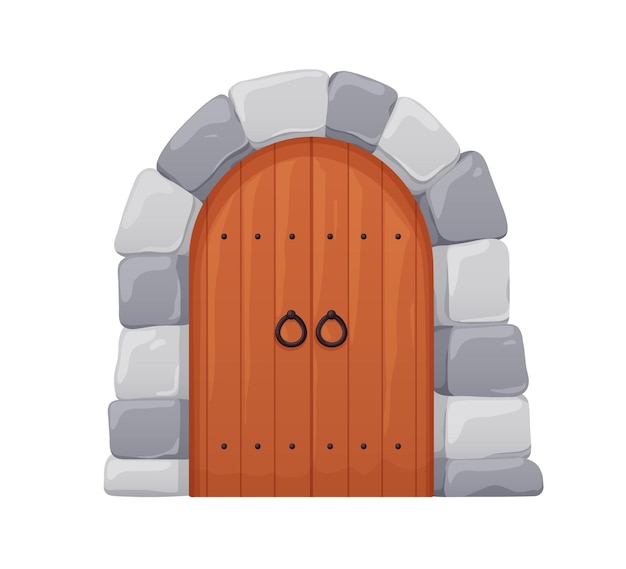The image is a detailed graphic artwork, possibly a cartoon rendering, of a medieval-era archway with a wooden double door. The arch around the door is constructed from alternating rectangular stones in a pattern of light gray and darker gray shades. The stone arch forms a U-shape, encasing the door. The door itself is made up of vertical wooden planks, totaling eight: six wider central panels and two narrower ones on each side. These planks are a brownish-orange color, each adorned with two large black bolt heads, one at the top and one at the bottom. The door opens in the middle, with two ring-shaped, dark brown handles situated on the innermost boards of each door panel. The entire scene is set against a white background, giving it a stark and clean appearance.